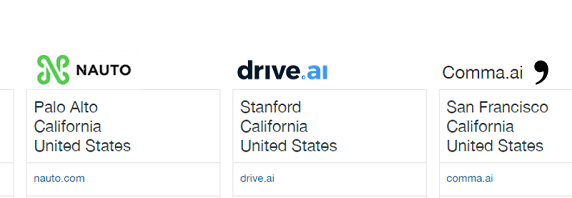The image features three distinct blocks, each with a detailed title and a light gray outline for definition. Each block contains three lines of text underneath its title, providing specific location information. Below the text, each block is complemented by a connected separator block displaying a hyperlink. 

- The first block is titled "NAUTO" and lists the location as "Palo Alto, California, United States." The corresponding web address is "NAUTO.com."
- The second block is titled "DRIVE.AI" and provides the location "Stanford, California, United States," with the associated web address "DRIVE.AI."
- The third block is labeled "COMMA.AI" and includes the location "San Francisco, California, United States," with the respective web address "COMMA.AI."

Each block is structured uniformly, creating a comprehensive and easily navigable presentation of information.